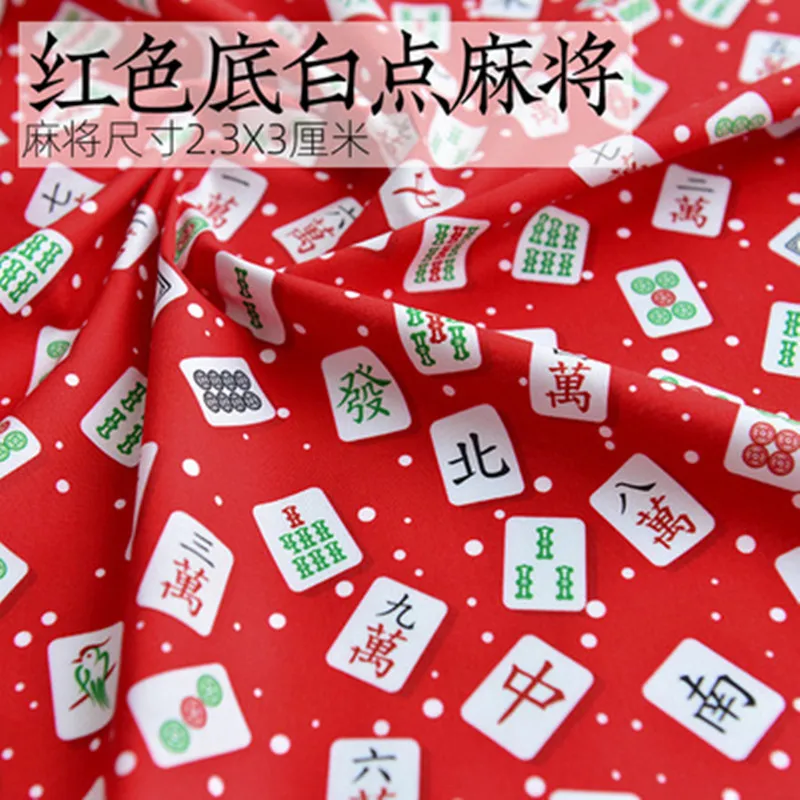The image depicts a brilliantly colored, deep red fabric adorned with numerous white, rectangular patches featuring rounded corners. Each patch contains intricate designs and an array of Japanese characters, reminiscent of Mahjong tiles, creating an intricate, patterned motif. Scattered across the red backdrop, between the rectangular patches, are white dots of various sizes. At the top of the fabric, there is what appears to be a clear label with large black Japanese characters, accompanied by additional smaller characters and numerals below, further enhancing the fabric's distinct Asian aesthetic.